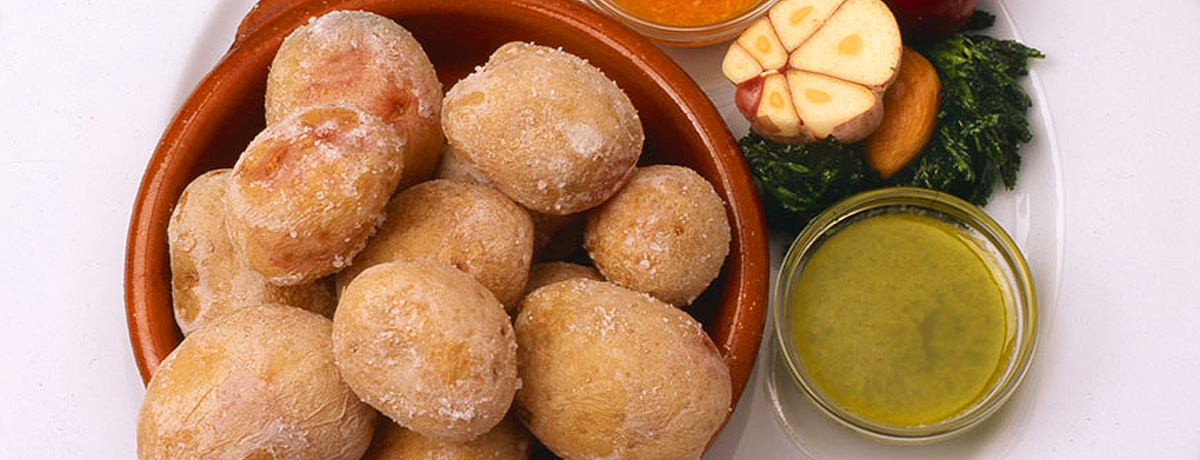The image depicts a top-down view of a food arrangement on a round white plate, which occupies most of the white background. To the left, there is a large dark brown bowl containing nearly round brown food items, which resemble small baby potatoes or possibly deep-fried pastries, each with a white topping. To the right of the large bowl, a small glass ramekin holds a green sauce. Above this ramekin, wilted greens and a half-cut head of garlic, showing six cloves, are placed together on the plate. A second smaller ramekin with red sauce can also be seen nearby, contributing to the diverse selection of food items displayed.